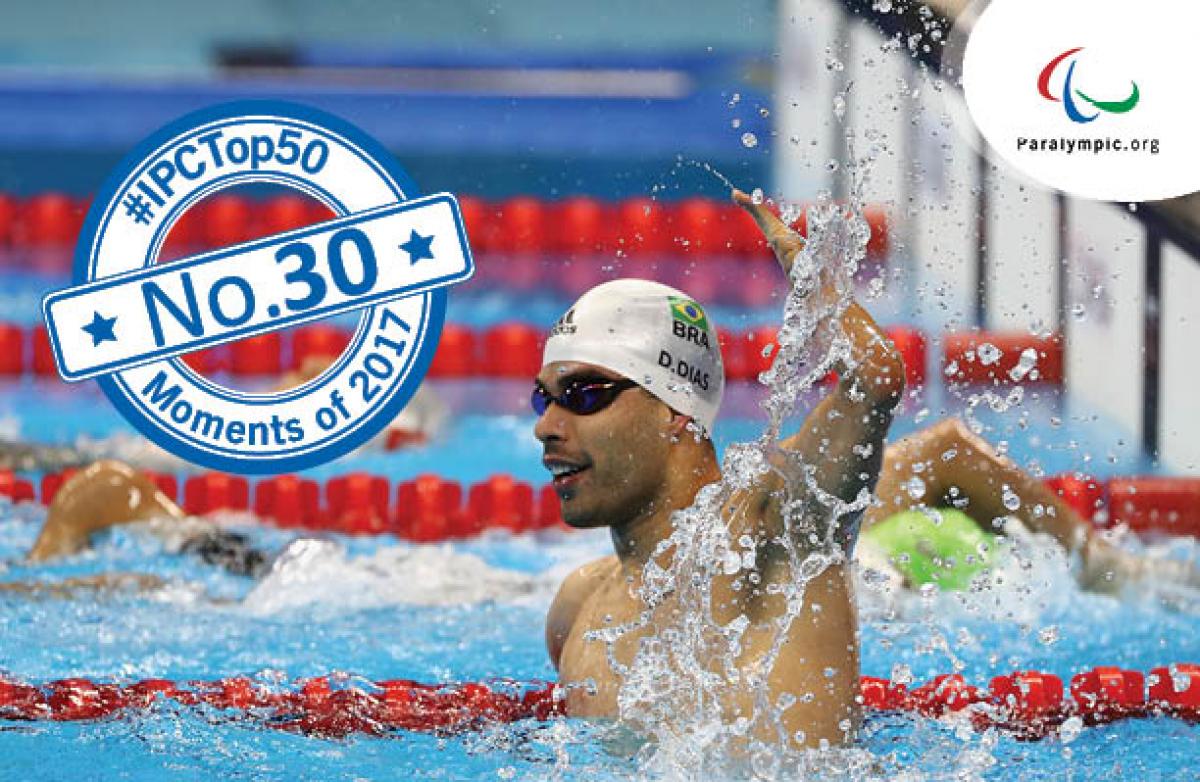This vibrant photograph captures the triumphant conclusion of a Paralympic swimming race, prominently featuring a confident athlete celebrating his victory. In the upper right corner, the Paralympic.org branding is displayed with a logo of three curves—red, blue, and green—set within a white circle. To the left, a banner marks this moment as one of the "IPC Top 50 Moments of 2017," specifically ranking it at number 30. The centerpiece of the image is a swimmer with a white cap bearing the Brazilian flag and the name "D Diaz." He raises his left arm in celebration, suggesting a victorious finish. His goggles reflect his focused determination. Other swimmers are seen trailing behind, still making their way towards the finish line. The pool's clear water and red lane dividers create a vivid backdrop for this moment of athletic achievement and pride.